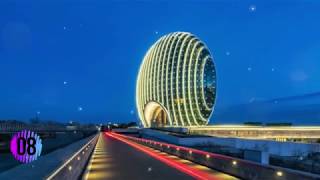The image is a small, digitally created rectangular scene set against a night sky in varying shades of blue, speckled with white stars. The primary backdrop features a horizontally rectangular format without any bordering edges. The lower left corner of the image displays a distinct purplish circle containing the black number "08." The central part of the image, leading upwards toward the middle, depicts an illuminated roadway adorned with yellow and red lines. To the center-right, there is a luminous, horizontal bar.

Dominating the scene are two golden circles, with the smaller enclosed within the larger, creating a striking focal point. These circles are crisscrossed by horizontal and vertical lines, forming an intricate grid pattern. The roadway appears to stretch into the distance, culminating in a large, reflective, bowl-shaped structure. This concave circle seems almost like a mirrored archway, bathed in light and accompanied by an entrance arch that remains partially obscured from view. The right portion of the structure is suffused with a yellowish glow, while the left side fades into darkness, possibly hinting at the silhouettes of buildings.